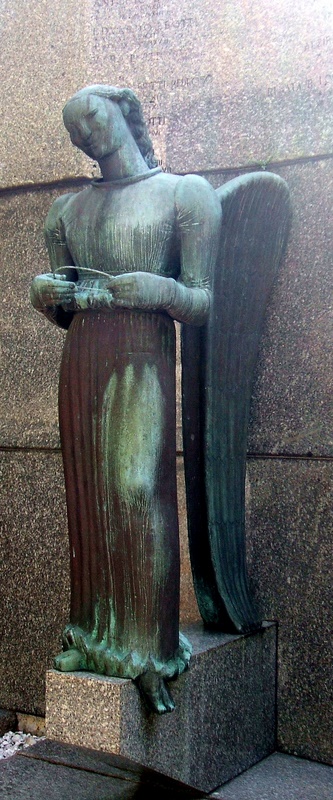The photograph is a tall, narrow portrait of a weathered bronze or copper statue, turned green over time, depicting a female angel with an intricate and serene demeanor. The angel is positioned against a backdrop of large, thick stone blocks extending from a stone wall, seemingly made of granite or a similar material. At the top center of the wall, an unreadable carving, possibly in Latin, adds a mysterious element to the setting.

The angel stands atop a small stone pedestal that extends outward from the wall. She has long, braided hair pulled back into a ponytail that cascades down her back. With finely detailed facial features, including narrow eyes, a straight nose, and a subtle smile, her head is slightly tilted to the right. The angel wears a high-necked, long-sleeved dress that bunches at her feet, descending gracefully to the base of the pedestal. Her right foot stands flat, while her left foot dangles off the edge, revealing two or three-toed hooves, adding an animalistic trait to her otherwise ethereal appearance.

Her arms are bent at the sides, holding a circular ring or halo in front of her waist. From behind her, a pair of long, folded angel wings emerge, almost reaching down to the pedestal, reinforcing her celestial nature. The camera captures the statue from an angled perspective to the left, accentuating the depth and detail of the scene.